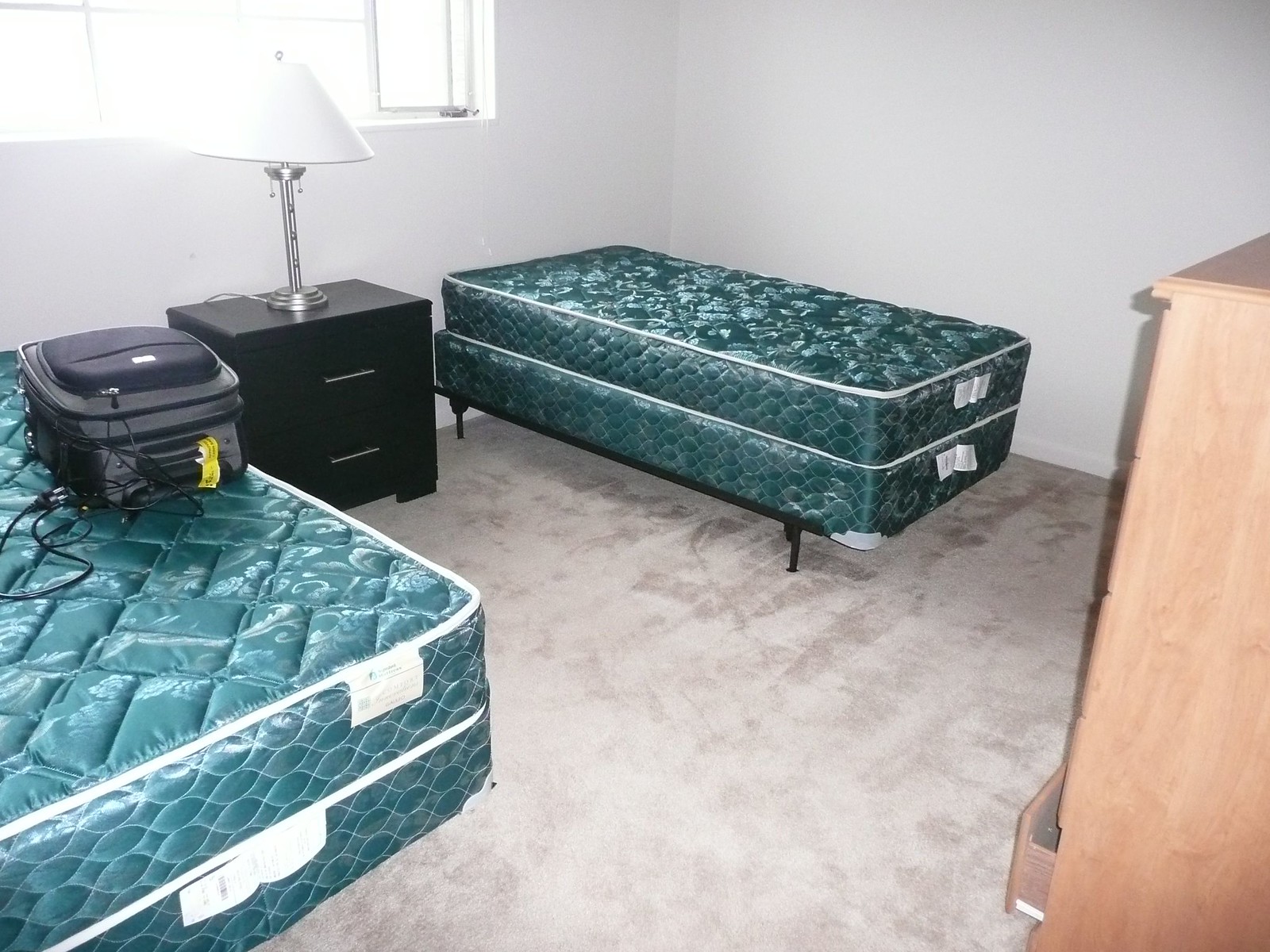The image depicts a well-lit, small bedroom viewed from the entryway. The room features two twin-sized beds without any sheets, pillows, or blankets, revealing just the green mattresses and box springs. The bed on the left side has a black suitcase on it, complete with cables, chargers, and a label from the airport. Positioned between the two beds is a fancy black nightstand, upon which sits an elegant lamp with an aluminum base and a white lampshade. The sunlight streams in through a couple of connected, uncovered windows, bathing the room in natural light. The flooring appears to be a beige-brown carpet. A wooden dresser drawer is slightly open in the bottom right corner of the image, casting a shadow. The room's white walls further enhance the bright, airy feel.